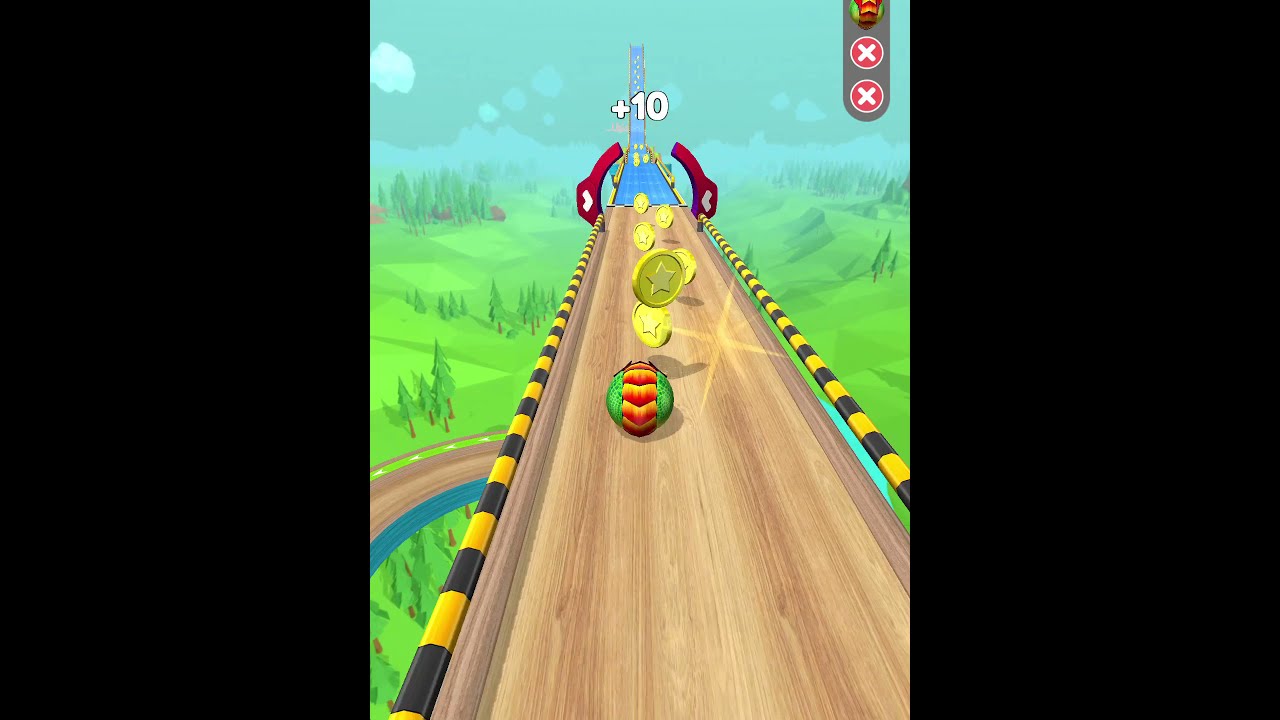This image is a screenshot from a cartoony, 3D-animated mobile video game. The main focus of the scene is a wood-textured racetrack with alternating yellow and black caution stripes along the guardrails. The racetrack stretches into the distance, transitioning into a blue, roller-coaster-like ramp. Below the track, there are grassy meadows and hills dotted with trees, adding to the natural background setting.

On the track, a sphere, possibly a lizard rolled into a ball, adorned with red and yellow stripes, is seen hurtling forward. The sphere is in the process of collecting yellow, star-marked coins, similar to those in Mario games. Each collected coin appears to add points, with a visible "+10" displayed in the middle of the image, directly above the track. In the distance, a red hoop can be seen, hinting at further challenges or obstacles ahead.

In the upper right corner, game interface elements are present, including an avatar and two red circles with white X's, likely indicating remaining lives or attempts. The entire scene is framed within a portrait-oriented view, with wide black margins on either side, emphasizing the central gameplay action.